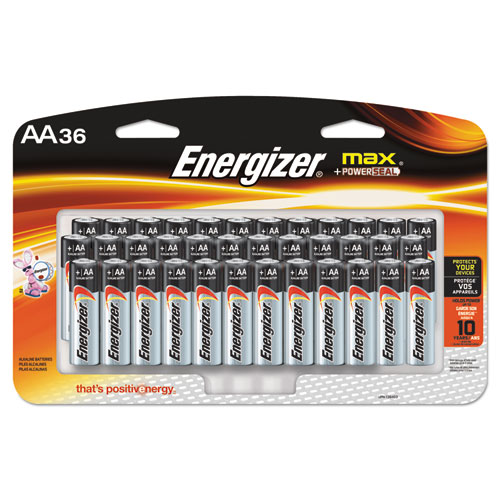The image displays a pack of Energizer AA batteries. The packaging is predominantly black at the top, adorned with vibrant orange and yellow lines that resemble glowing, hot metal. At the top left corner, "AA36" is prominently featured, indicating the battery type and quantity. The package is designed with two unique white holes, which are a cross between a triangle and a rectangle, allowing it to be hung on a shelf.

The brand name "Energizer" is written in white italic text, and just below, in bold yellow text, it reads "Max Plus Power Cell." The package showcases three neat rows of batteries, each row containing a dozen batteries. The batteries themselves are designed in a sleek gray and black color scheme with a distinctive red and gold stripe on the side.

On the left side of the packaging, the iconic pink Energizer Bunny is depicted beating its drum. At the bottom, the phrase "Positive Energy" is prominently displayed, reinforcing the brand's messaging. There is also some additional text on the right side of the package, which is too small to decipher in the image.